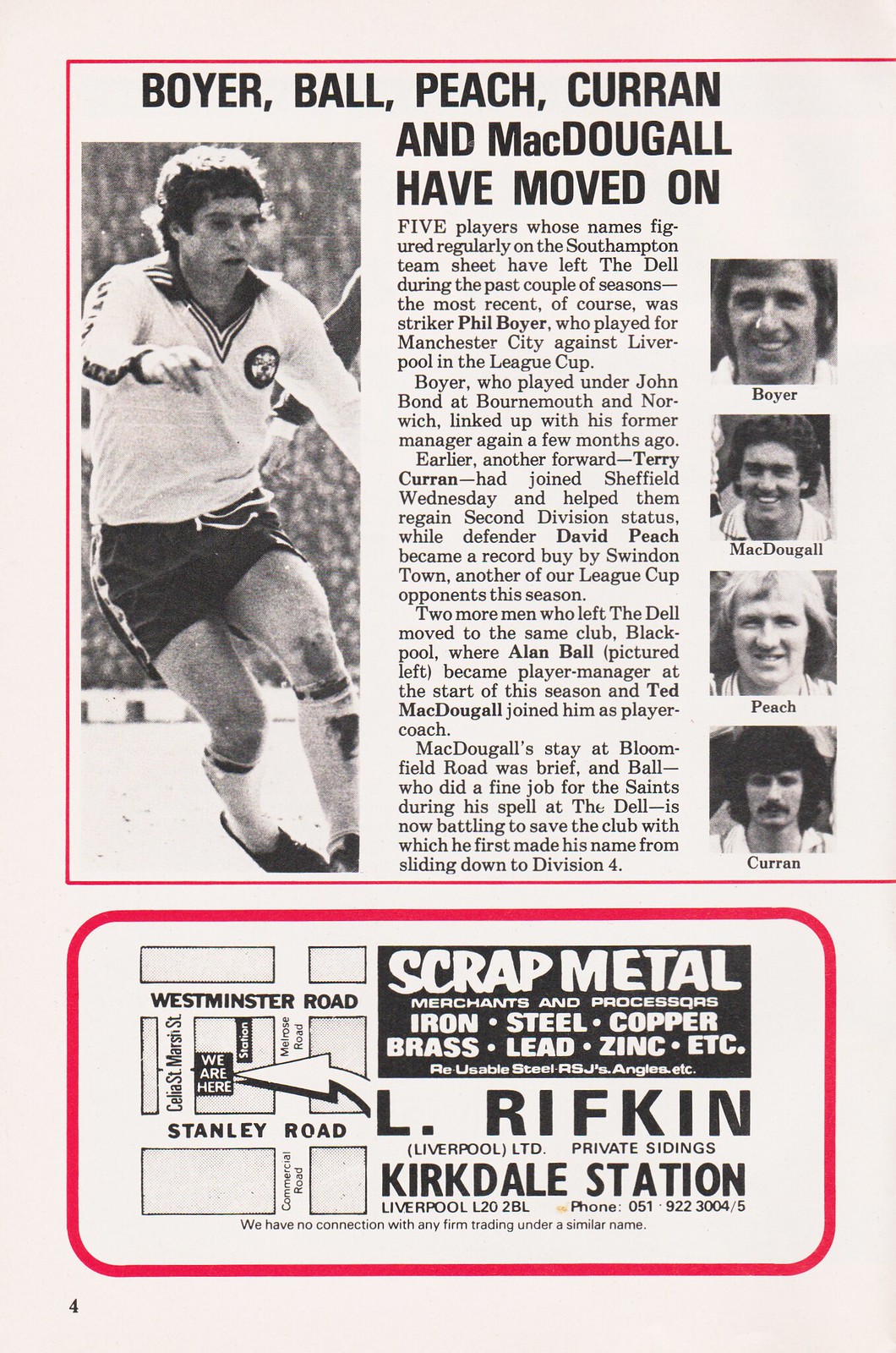The image depicts a page from an old magazine, showcasing a detailed article about five English football players—Boyer, Ball, Peach, Kern, and MacDougall—who have left their team. The page is taller than it is wide, with an off-white to grayish background and pinstriped red borders framing the content. The top section features a bold headline, "Boyer, Ball, Peach, Kern, and MacDougall Have Moved On," followed by four paragraphs explaining why each player left and their backgrounds. On the left, there is a full-length rectangular photo of Ball, dressed in a long-sleeve white jersey, dark shorts, and white socks, captured in action on a soccer field with a stadium in the backdrop.

Adjacent to the text, from top to bottom, are headshot photos of Boyer, MacDougall, Peach, and Kern, each labeled accordingly. The bottom section of the page contains a rectangular advertisement with a red outline and beveled edges. Inside, a black rectangle with white text reads, "Scrap Metal Merchants and Processors: Iron, Steel, Copper, Brass, Lead, Zinc, etc." Further details include: "L. Rifkin, Kirkdale Station, Liverpool L202BL," along with a phone number and a disclaimer about no affiliation with similar-named firms. To the right, a tiny road map illustrates the company's location, marked by an arrow indicating "We are here," and highlighting nearby streets, Stanley Road and Westminster Road. The lower left-hand corner of the page is marked with the number "4."